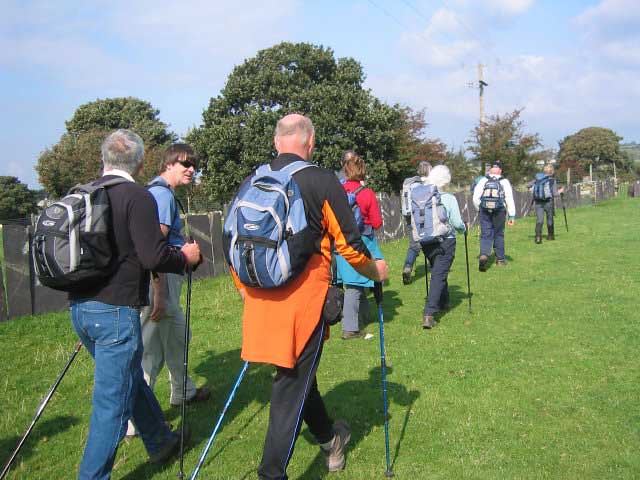In this outdoor photo, a group of older individuals, identifiable by their gray hair, is captured hiking in either a single or double file through a vibrant green field. Each person is equipped with a pair of blue or black walking sticks and a backpack, which are predominantly shades of blue, gray, and black. They are all dressed in dark slacks or jeans and most are wearing long-sleeved shirts, appropriate for warm weather, though one man sports a blue t-shirt with khaki pants. A noteworthy detail is the variety in backpack colors, and everyone seems to be wearing sturdy hiking boots. On the left side of the image runs a five-foot-high mesh fence, beyond which trees can be seen. The scene is set under a sunny sky dotted with white clouds. Prominent individuals in the image include two older men at the forefront – one with a black long-sleeved shirt, blue jeans, and a gray backpack, the other with a black and orange long shirt and a large blue backpack. A middle-aged man with dark hair and sunglasses, dressed in a blue shirt and khaki pants, appears to be observing the group. Additionally, a woman in a blue t-shirt with white hair and navy blue pants carries her walking sticks diligently. Off in the distance, silhouettes of more hikers can be spotted, blending into this serene and organized adventure. A notable landmark in the background is a tall pole that possibly holds a flag, adding a touch of character to the picturesque setting.